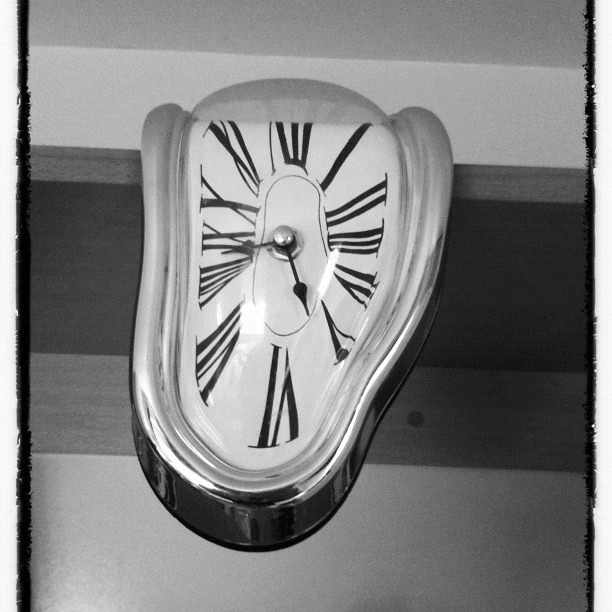This detailed black and white surrealist image features a melting clock with a shiny silver frame, hanging precariously off the edge of a gray wooden ledge. The deformed clock face, seemingly drooping like a slab of steak, is warped as it hangs over the side. The clock's numbers, displayed in Roman numerals, enhance its elegant yet surreal appearance. The clock hands, set to 5:45, appear immobile, suggesting the clock is stuck at this specific time. The overall tone and composition of the image create a sense of eerie distortion, characteristic of a surrealist piece.